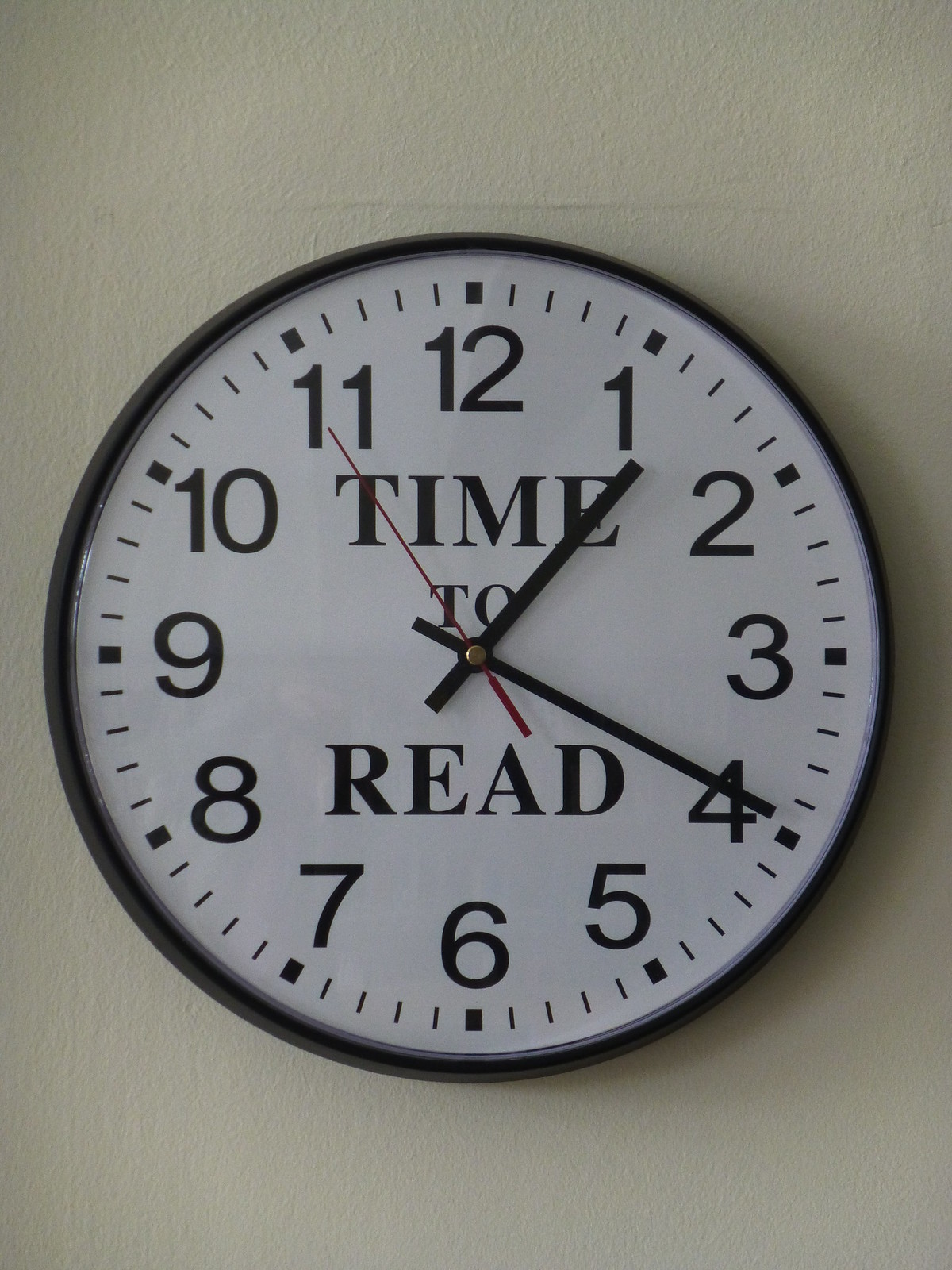This photograph features a classic analog wall clock, suspended against a plain white wall, illuminated by natural daylight. The clock, powered by a battery, displays traditional English numerals from 1 to 12, with minute and second markers encircling the outer edge. At its center, the phrase "Time to Read" is prominently displayed. The second hand is a striking red, while the hour and minute hands are black. The overall color scheme of the clock is a contrast of white and black, with the white serving as the background and the black detailing the numerals and lettering.